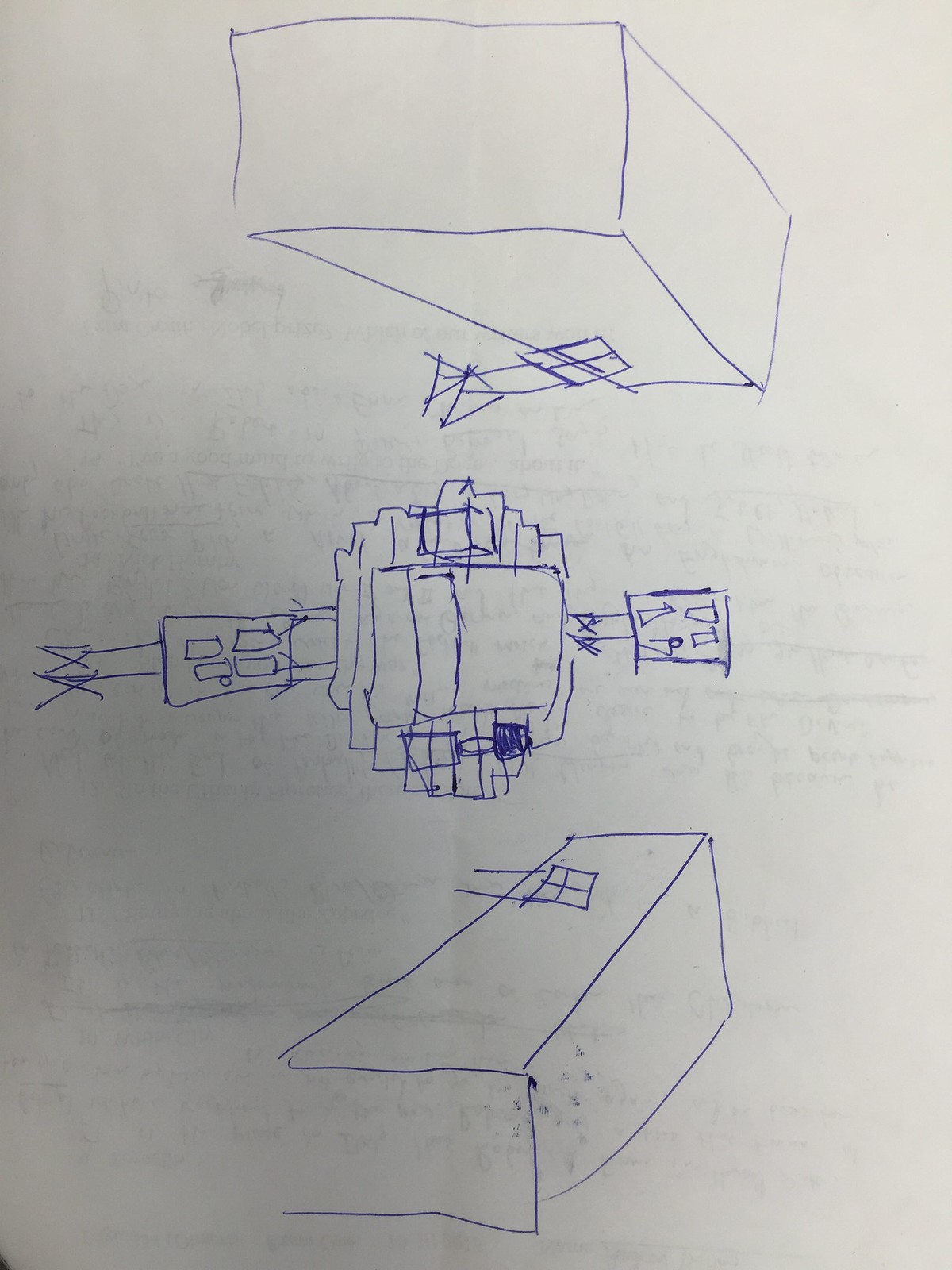This intriguing sketch, rendered in blue ink using a blue pen, prominently features a central figure that could be interpreted as either a robot or a microphone. The focal point of this figure is a TV screen-like element situated in its middle, adding to its enigmatic and futuristic appearance. The intricacy of the inking and the imaginative design make this piece a captivating example of inventive sketch artistry.